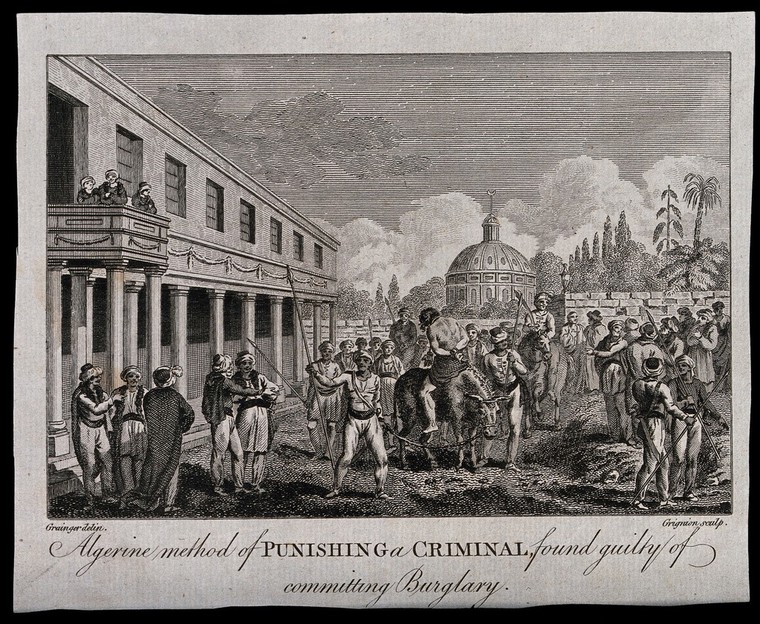The image displays a detailed black-and-white illustration, possibly from an old book or historical record, with a black and white border. The caption in cursive reads: "Algerine method of punishing a criminal found guilty of committing burglary," except for the words "punishing" and "criminal," which are in a regular font. The illustration features a man bound and blindfolded, positioned backwards on a horse, shirtless and dressed only in a waist cloth. His hands are tied behind him. Surrounding him are men armed with spears, creating a tense atmosphere. This scene unfolds in a courtyard with a large crowd watching, adjacent to a two-story building with white pillars and a balcony filled with onlookers. The background reveals more architectural details, including a cylindrical building with a pole on top, reminiscent of a dome, and additional elements like clouds and trees near a stone wall. The attire of the figures suggests a Middle Eastern setting, with traditional headbands and long garments similar to those found in Saudi Arabia.